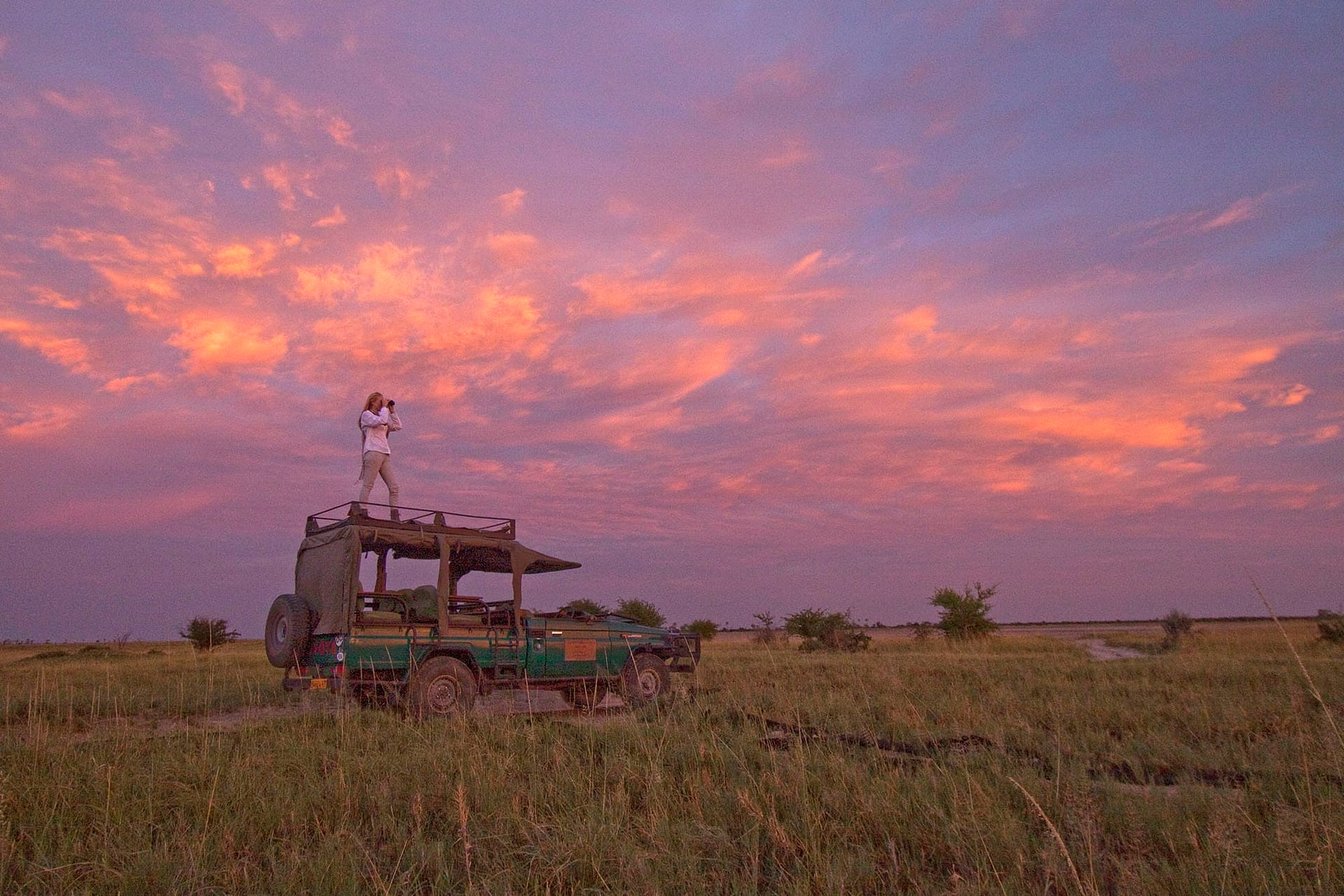In this vibrant sunset scene set in a vast, open field that resembles a desert or savanna, a green safari truck with open sides stands out against the landscape. The truck is navigated along a dirt path through tall, somewhat scorched grass interspersed with sparse bushes and trees. Atop the vehicle, a woman dressed in a white shirt and tan pants, likely a tourist, stands with a camera, capturing or perhaps savoring the moment. The sky is ablaze with stunning hues of orange, pink, and purple, with wisps of blue peeking through, reminiscent of both cotton candy and a gentle fire. The scene, suggestive of an African safari, is filled with the serene beauty of nature at either sunrise or sunset.